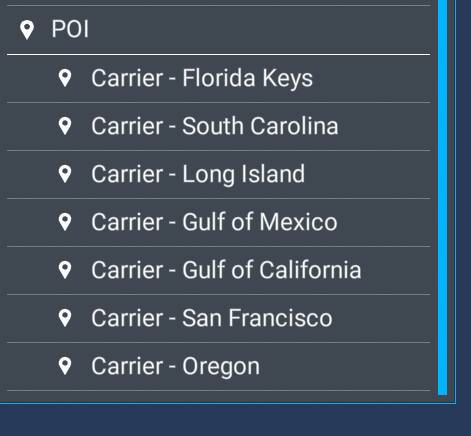The image displays a detailed list of locations under the title "POI." Positioned at the top is the title "POI," accompanied by a white app pin icon to the left. Beneath this title, seven distinct carriers are listed, each prefaced by the same white map pin icon and labeled with "carrier." Following "carrier" is a hyphen indicating the specific location of each entry. The locations included are:

1. Florida Keys
2. South Carolina
3. Long Island
4. Gulf of Mexico
5. Gulf of California
6. San Francisco
7. Oregon

Each of these carriers is separated by a thin gray line. The background of the list is a dark gray color. To the right side of the list, there is a vertical blue line, and a blue outline frames the entire dark gray square, providing a neat and organized appearance to the layout.